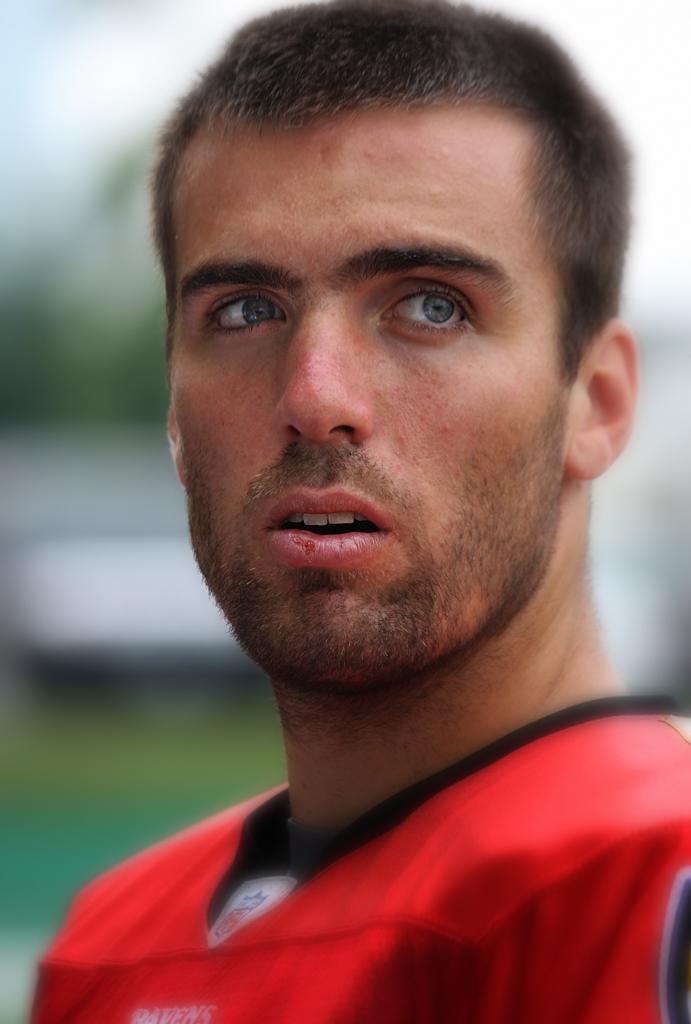This image is a close-up photograph of NFL quarterback Joe Flacco during his younger years, sporting a red Ravens practice jersey with black trim around the collar. An NFL logo tag is visible at the neckline, and there’s a hint of a blue number on the shoulder pads. Joe’s appearance is marked by his closely cropped dark brown hair, dark eyebrows, and striking blue eyes. His facial features include a short, stubbly mustache and beard, as well as slight acne and a small scab on his lip. He is facing left at a three-quarter angle, with his eyes looking off into the distance above his left shoulder, and his mouth slightly open. The background is heavily blurred, depicting what appears to be a grassy athletic field, some benches, and a faint outline of the sky. Trees and a white structure are also vaguely visible in the background.